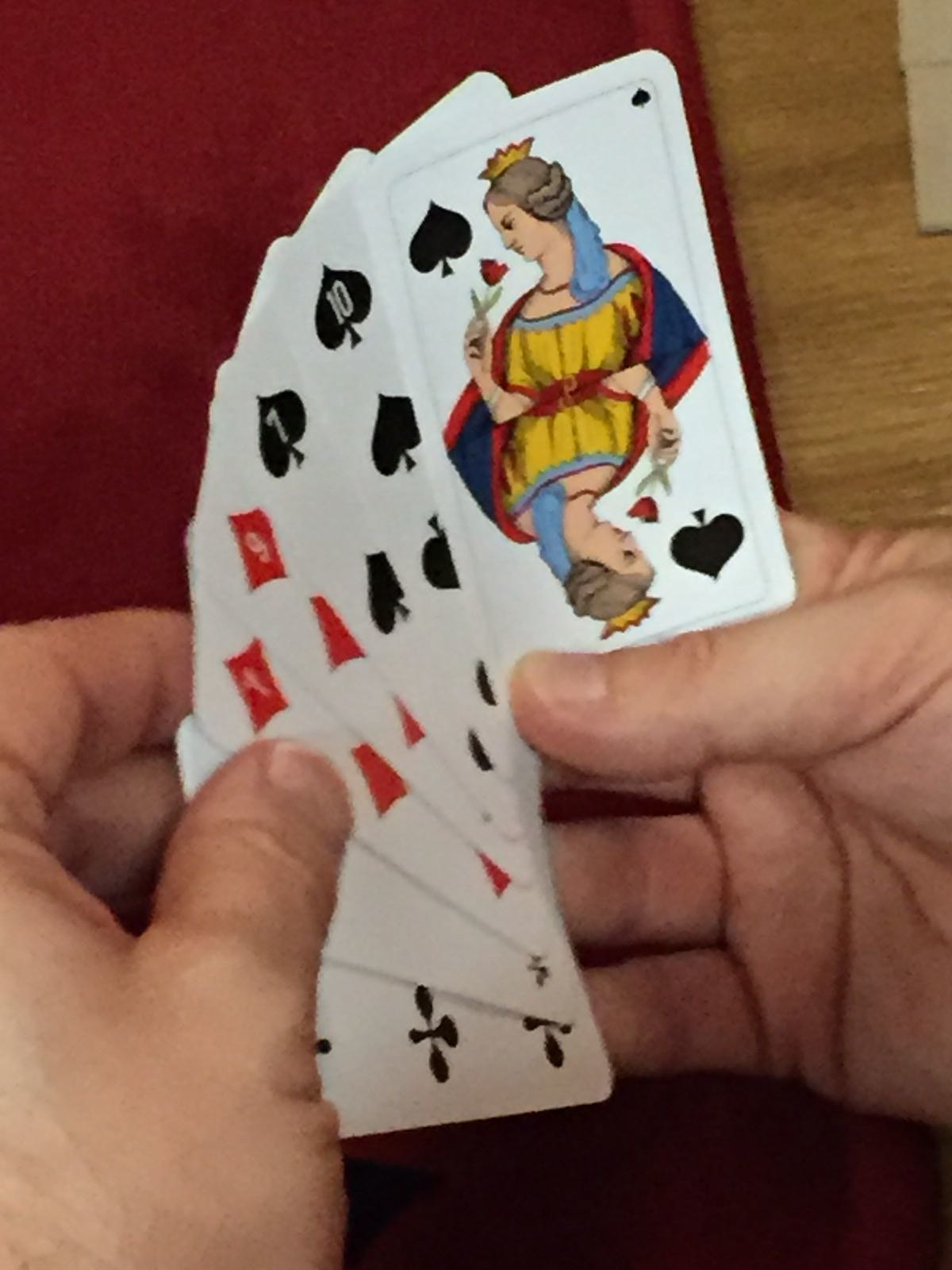In this vibrant color photograph, a person is holding a fan of playing cards in their hand. The visible cards include the Queen of Spades, the Ten of Spades, the Seven of Spades, the Nine of Diamonds, and the Seven of Diamonds. The remaining two cards, both Clubs, are partially obscured by the person’s thumb. The composition is set against a rich red felt surface, hinting at a gaming table. To the right of the hand and cards, a wooden table edge is visible with a small notepad resting atop it, possibly used for keeping score. The Queen of Spades in the hand stands out with her detailed depiction: she has brownish hair, adorned with a gold crown from which a blue scarf flows. She’s elegantly dressed in a golden gown with a red sash, holding a flower in her left hand. A blue shawl with a red border drapes between her arms, adding to the intricate design of the playing card.